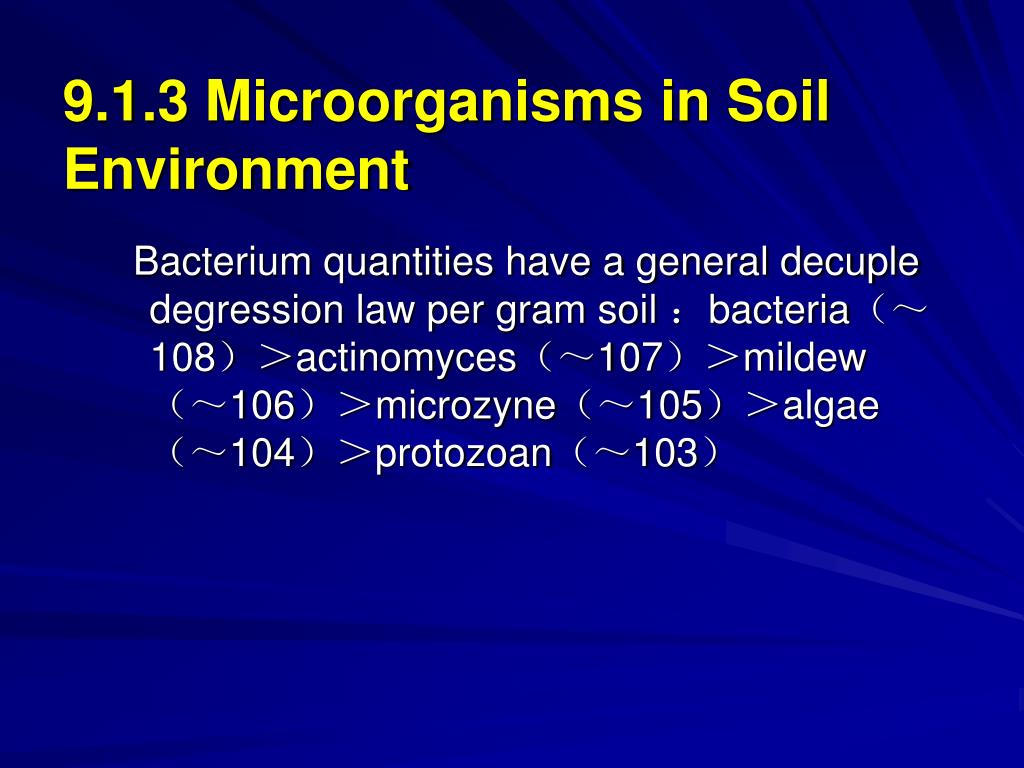The image features a PowerPoint slide with a variegated blue background transitioning from darker to lighter shades. The blue background has an intricate design, with angular streaks radiating from the center middle, varying in shades from dark to light blue. At the top left of the slide, yellow text reads "9.1.3 Microorganisms and Soil Environment." Centered beneath this, white sans-serif text states, "Bacterium quantities have a general decuple degression law per gram soil," detailing the hierarchy of microorganism quantities in soil: Bacteria (10^8) > Actinomyces (10^7) > Mildew (10^6) > Microzyme (10^5) > Algae (10^4) > Protozoan (10^3). This slide is likely from an educational presentation or study, illustrating the relative abundance of different microorganisms in soil.